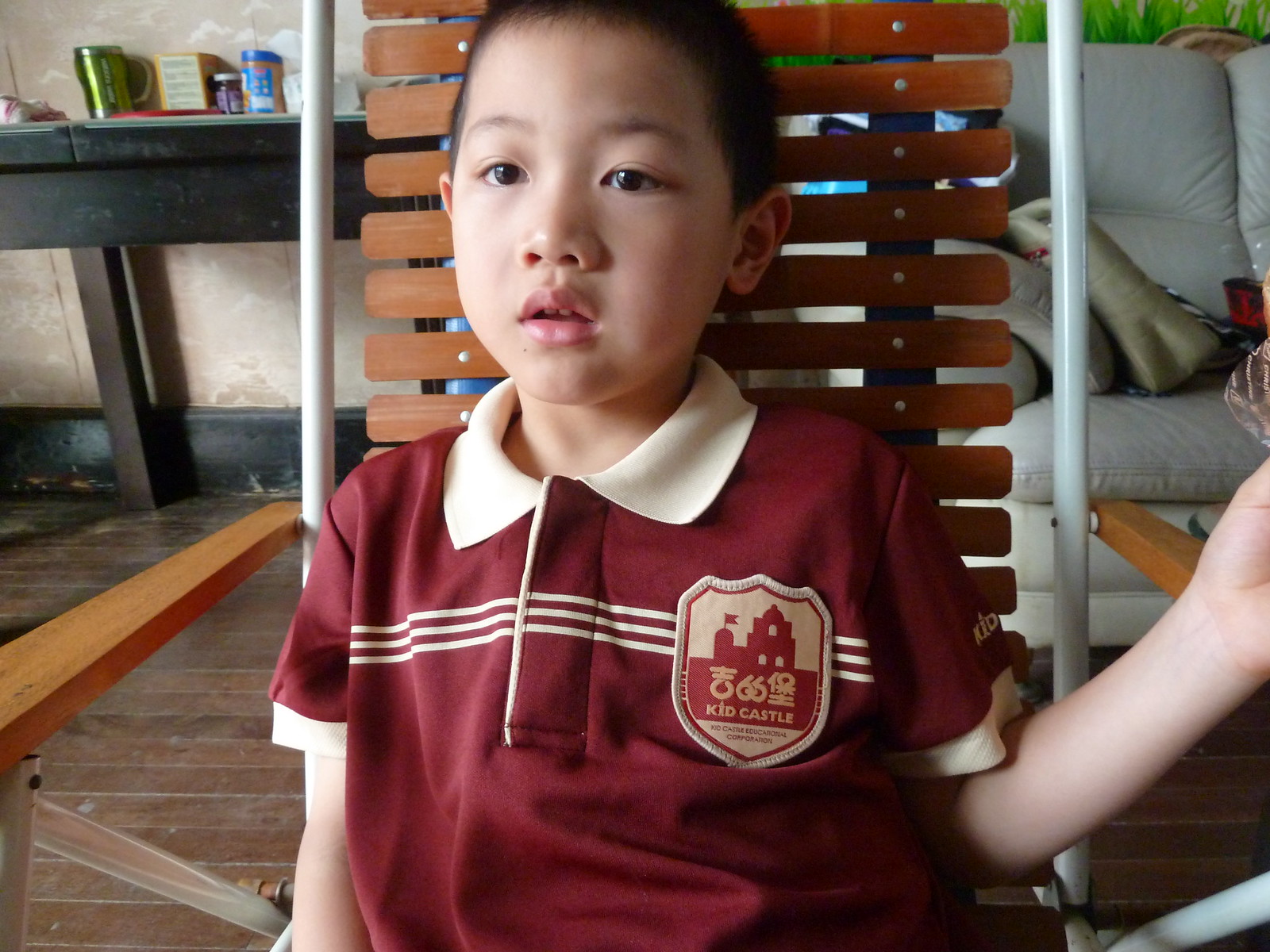The image depicts a young East Asian boy, dressed in a maroon and beige school uniform polo with a badge that reads "Kid Castle Educational Corporation" featuring a shield logo with a castle outline. He is sitting in a beach chair with horizontal wooden slats and a white metal frame. The room has hardwood floors and is furnished with a tan wallpapered wall having a black border at the bottom. To the boy’s right, there's a white sofa adorned with green pillows, along with a leather purse and possibly a toy on top. To his left, a black table against the wall holds various items, including a mug, a pill bottle, a jar of peanut butter, and a bag of marshmallows. The boy faces the camera with his mouth slightly open, creating an inviting indoor scene.